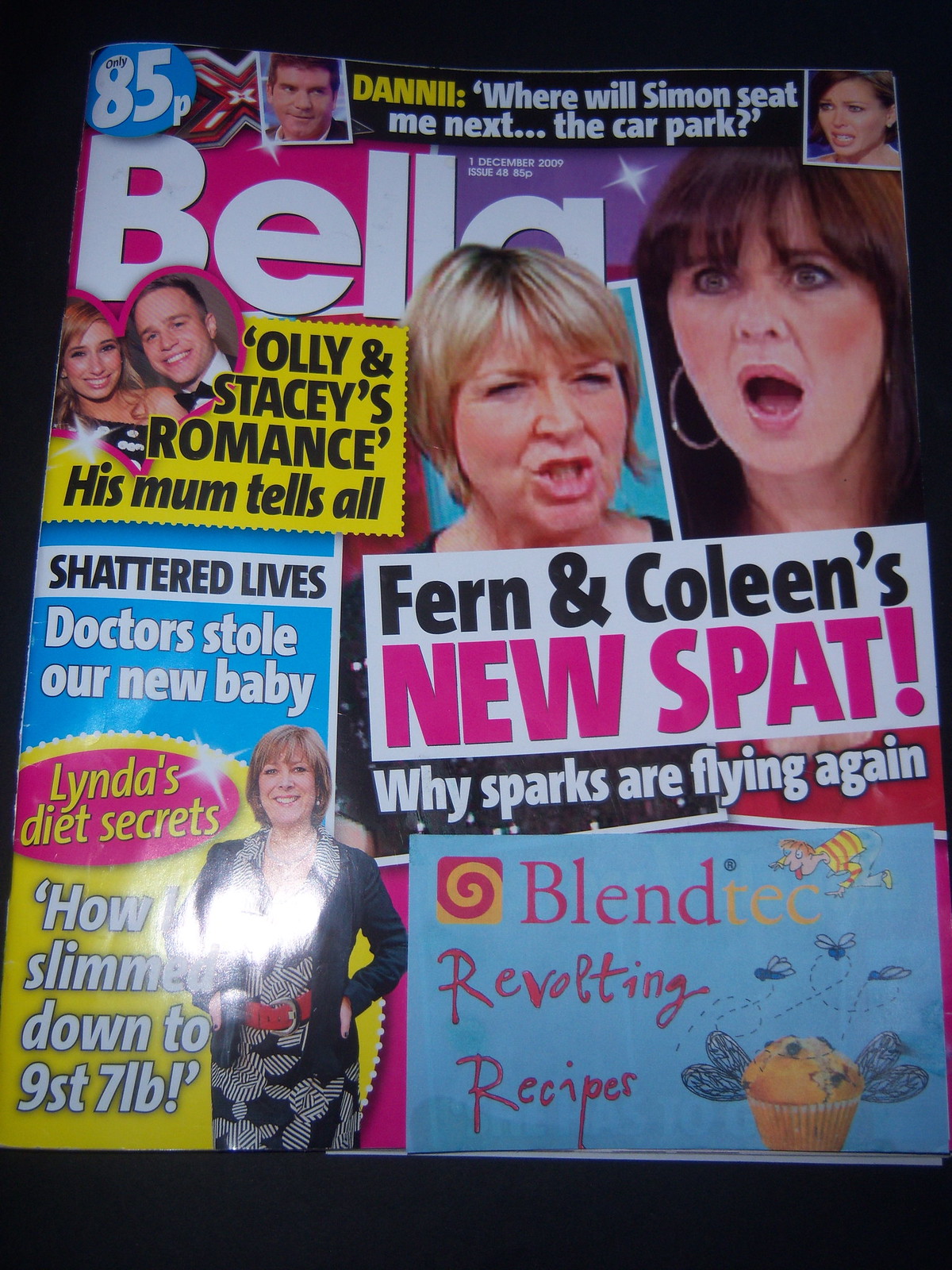Against an all-black background, the photograph showcases the bustling cover of the December 1st, 2009 issue of the British magazine "Bella," priced at 85 pence. Central to the design is an array of shocked and expressive faces of various individuals, highlighting the gossip-centric content of the magazine. Prominent headlines include “Ollie and Stacey's romance, his mum tells all,” nestled within a pink heart design, and “Fern and Colleen's new spat, why sparks are flying again,” accompanied by images of two women with open mouths—one blonde and one brunette. A dramatic headline reads, “Shattered lives: doctors stole our new baby,” and another notes “Linda's diet secrets: how I slimmed down to nine stone seven pounds.” At the bottom right, a provocative section titled "Blendtec Revolting Recipes" features an image of a blueberry muffin surrounded by illustrated flies and a small cartoon character. The vibrant color scheme predominantly features white, fuchsia, purple, yellow, and bright blue, reflecting the magazine's dynamic and eye-catching style.